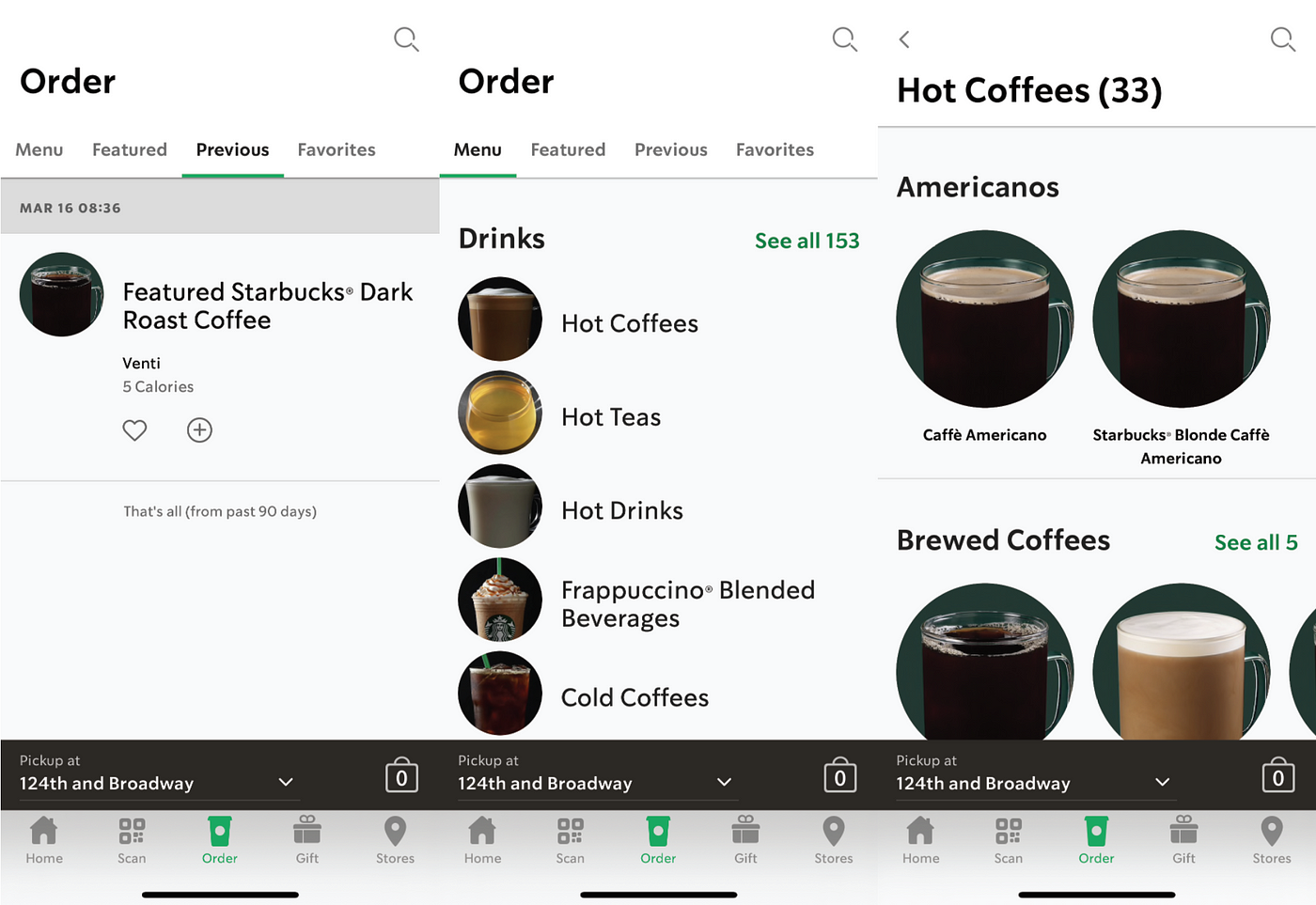The image features a digital interface with three screens displayed side-by-side. 

1. **Left Screen: Order Section**
   - The screen titles "Order" followed by submenu options: "Menu," "Featured," "Previous," and "Favorites." 
   - The "Previous" tab is highlighted with a green underline.
   - Below the highlighted tab, there is a gray box containing the date and time "March 16th, 08:36" along with a photo of a dark liquid in a clear mug.
   - The text under the photo reads: "Featured Starbucks Dark Roast Coffee, 25 calories," accompanied by icons of a heart and a circle with a plus sign.
   - A note at the bottom states, "That's all from past 90 days."
   - The bottom of the screen displays a black box with the text "Pick up at 124th and Broadway," together with a downward-pointing arrow and a shopping bag or briefcase icon with a zero in the middle.

2. **Middle Screen: Categories**
   - There is no specific text provided for the middle screen beyond categories like "Hot Coffee," "Hot Tea," "Hot Drinks," "Frappuccino Blended Beverages," and "Cold Coffee."
   - Each category is symbolized by an icon or thumbnail, positioned to the left of the text.

3. **Right Screen: Drinks Section**
   - The screen is labeled "Drinks CR 153."
   - This section lists different beverage options with corresponding icons or thumbnails:
     - Hot Coffee
     - Hot Tea
     - Hot Drinks
     - Frappuccino Blended Beverages
     - Cold Coffee
   - This screen also includes a pickup location note: "Pick up at 124th and Broadway."

The entire interface seems designed for easy navigation and selection of previous orders, featured items, and categorized drink options.